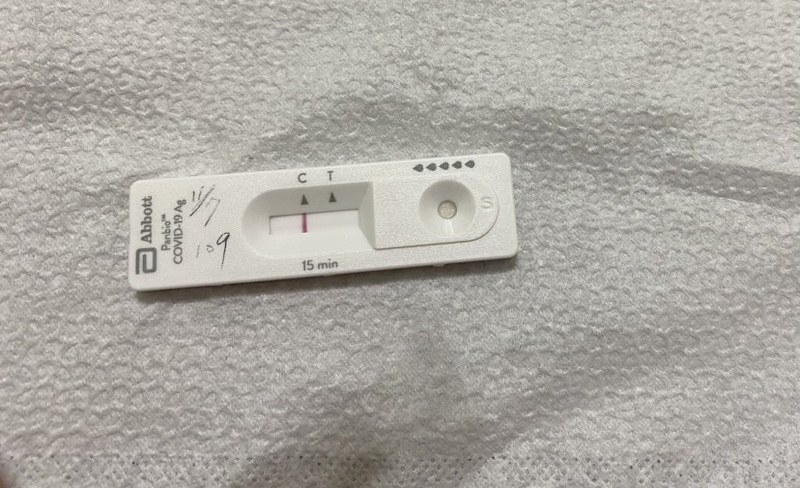The photograph, taken in landscape orientation, captures a COVID-19 test kit leaning against a crinkled paper, which appears to be either paper towel or toilet paper. The textured paper extends from the bottom left to the bottom right, marked with numerous tiny black dots. The paper's crinkled surface features noticeable indentations.

The COVID test kit itself is oriented horizontally from left to right. On the left side of the test, the Abbott logo is visible, followed by the text "PANBIO™ COVID-19 Ag." Below this branding, there is handwritten text that reads "11/7, 109," likely indicating the date and time the test was taken—November 7th at 1:09. The test has a control line labeled "C," marked with a triangle and a thick red line, and a test line labeled "T," marked with a triangle but no line, indicative of a negative result. It also features the instruction "15 min" at the bottom, indicating it is a 15-minute COVID test.

In the upper right corner of the image, five teardrop-shaped dots are aligned from left to right. The right side of the test kit shows an opening with a circular area in the middle, allowing a view through to the crinkled paper background. Beside this opening, the letter "S" is visible.